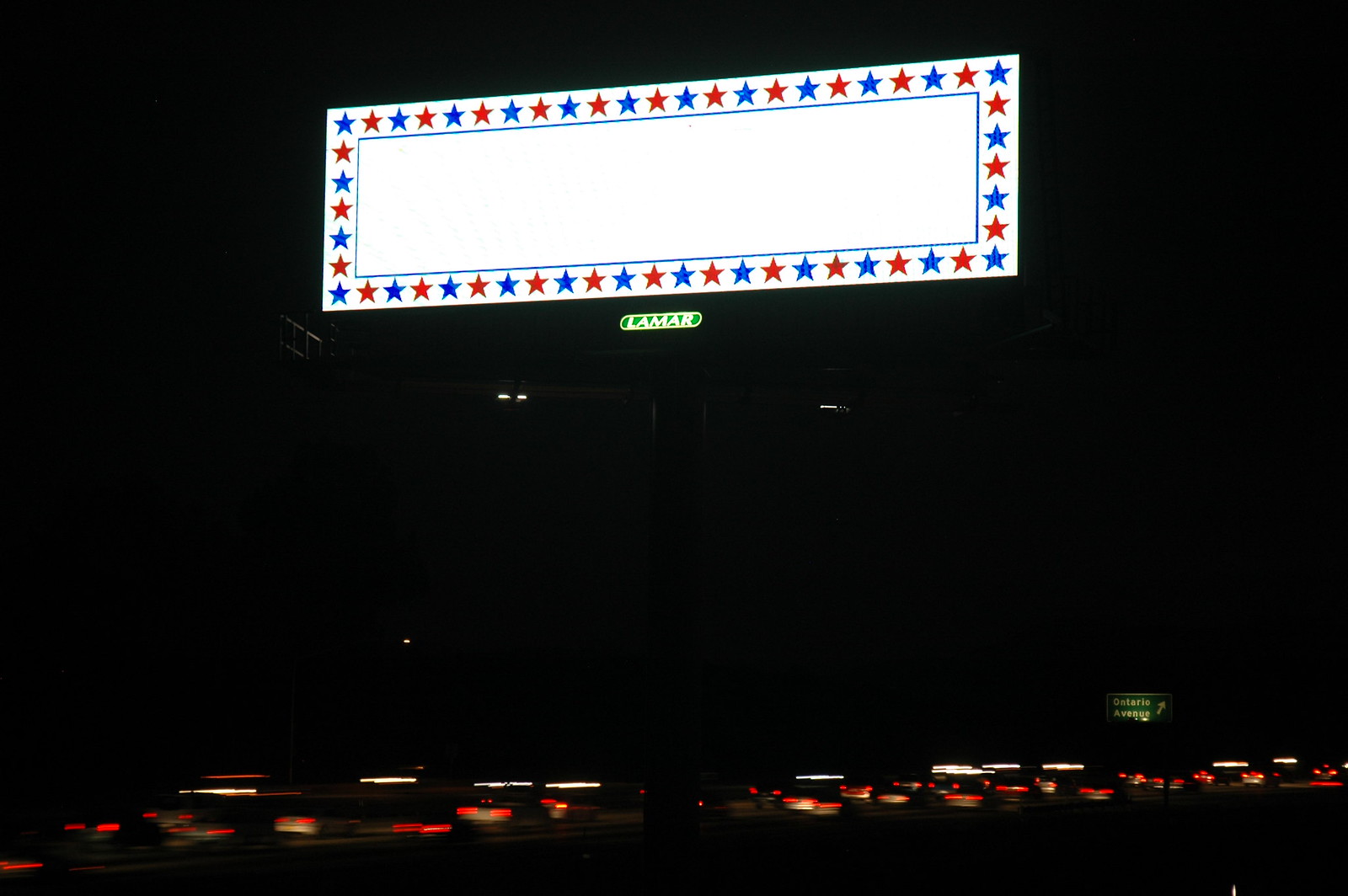A first-person perspective nighttime photograph captures a fully illuminated billboard from a slightly elevated roadside position, possibly from a parked car. The billboard is positioned on a singular pole and features a prominent white LCD-lit screen. Encircling the billboard is a vibrant border of alternating blue and red stars, creating a patriotic aesthetic. Inside this border lies a thin blue rectangle, framing the otherwise blank white background of the billboard.

The night sky forms a dark backdrop, enhancing the bright display. Below the billboard, occupying the lower third of the image, there’s visible motion blur from the headlights and taillights of moving cars on a highway, creating streaks of red and white light. To the right of the busy road, a green directional sign with white lettering is partially discernible. The sign includes an upward-pointing arrow indicating a right turn. Although slightly difficult to make out, the sign possibly reads “Gataro Avenue,” with “Avenue” being more legible.